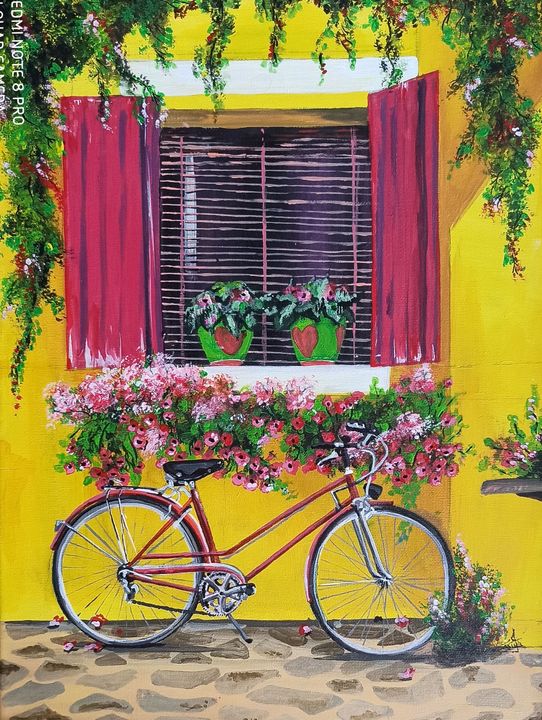This vibrant and cheerful illustration in portrait mode showcases the exterior of a brightly colored yellow building. The focal point of the image is a classic red bicycle with hand brakes and a black seat, parked against a tan and gray cobblestone pavement directly beneath a charming window. The window features open red shutters and horizontal blinds, flanked by green hanging plants. The windowsill is adorned with two green pots decorated with red hearts, filled with pink flowers and green leaves, while additional pink, red, and white flowers and greenery stretch horizontally below the window. The bright and colorful scene is complemented by vines cascading down the side of the building and scattered red and pink petals on the ground, adding to the illustration's lively and picturesque ambiance.